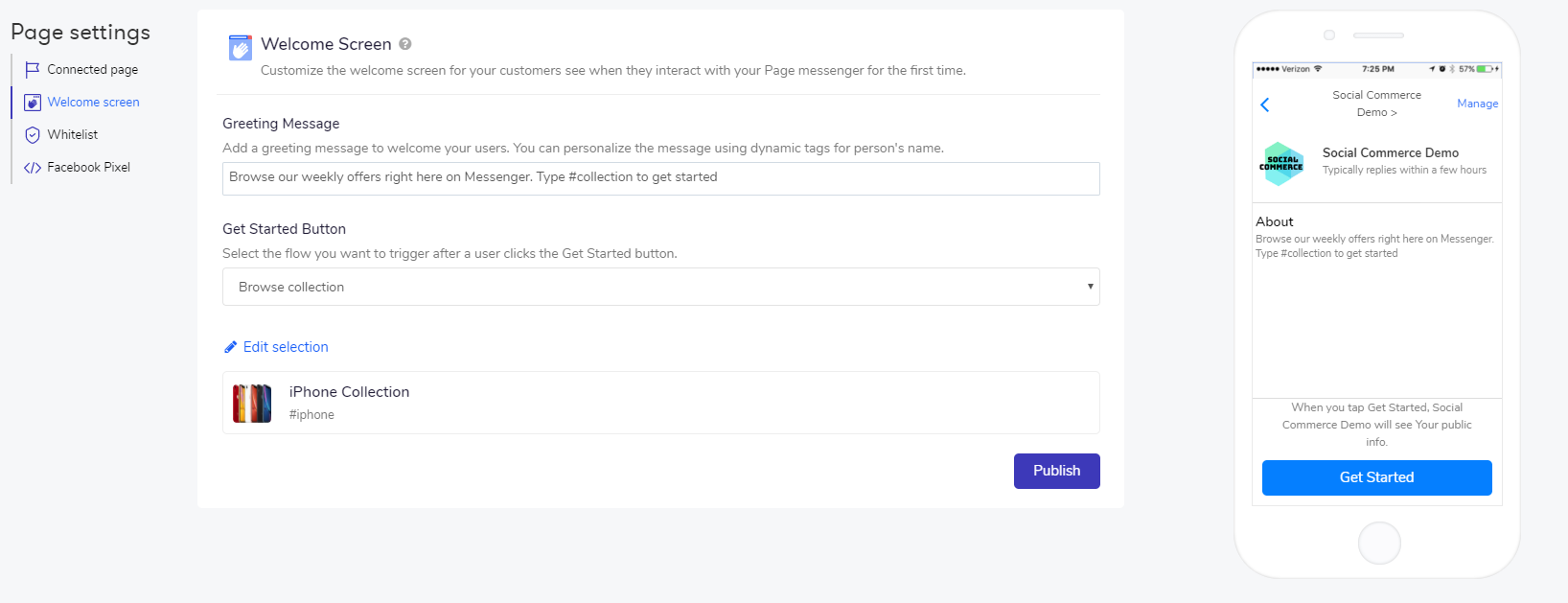**Detailed Caption:**

This image is a screenshot of the page settings for computers, showcasing various configuration options. In the left pane, titled "Page Settings," a list of settings is displayed, each accompanied by a distinctive icon. The first item, "Connect Page," features an icon of a flag. Next, "Welcome Screen" is paired with a browser icon. The third item, "Whitelist," includes an icon of a shield with a checkmark inside it. Lastly, "Facebook Pixel" displays an icon with two arrows—a left-pointing arrow, a slash, and a right-pointing arrow.

In the main body of the browser, detailed settings for the "Welcome Screen" are prominently featured. This section allows customization of the welcome screen that users will see when they first interact with your page via Messenger. Following this is the "Greeting Message" section, where you can personalize the greeting message visible to users. The "Get Started Button" section allows you to browse and configure a collection of buttons that are triggered when a user clicks the "Get Started" button. Below these options is an "Edit" section. 

At the far right corner, a purple box with the label "Publish" can be seen. To its right is an image of a cell phone displaying a social commerce demo, complete with a "Get Started" blue button at the bottom.